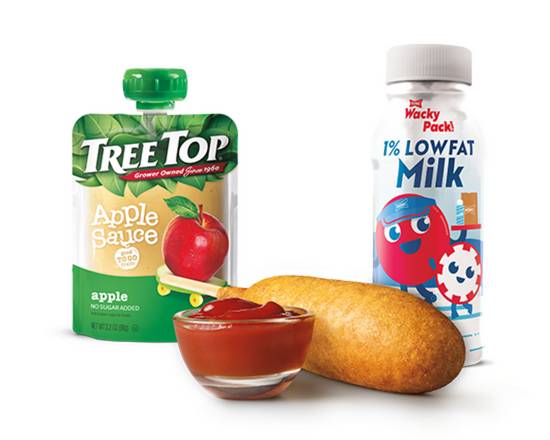This is a meticulously arranged group photo showcasing various food items, ideal for a child’s lunch. Centrally positioned is a corn dog with a tanned, crisp outer layer on a popple stick, paired with a small glass bowl containing vibrant red ketchup. To the left of the corn dog is a packet of Tree Top applesauce, featuring a green top and bottom with white text on a beige center that partially reveals the applesauce inside. The packet is adorned with an image of an apple. On the right side of the image is a small white bottle of Wacky Pack 1% low-fat milk, decorated with blue text and a cartoonish red figure resembling a chip or character, adding a playful touch. The items are set against a pure white background, emphasizing the natural colors of the applesauce, the corn dog, and the milk, making the food appear even more appealing. This carefully composed image likely serves as a suggestion for a wholesome kid's meal option, possibly featured on a promotional website or advertisement.